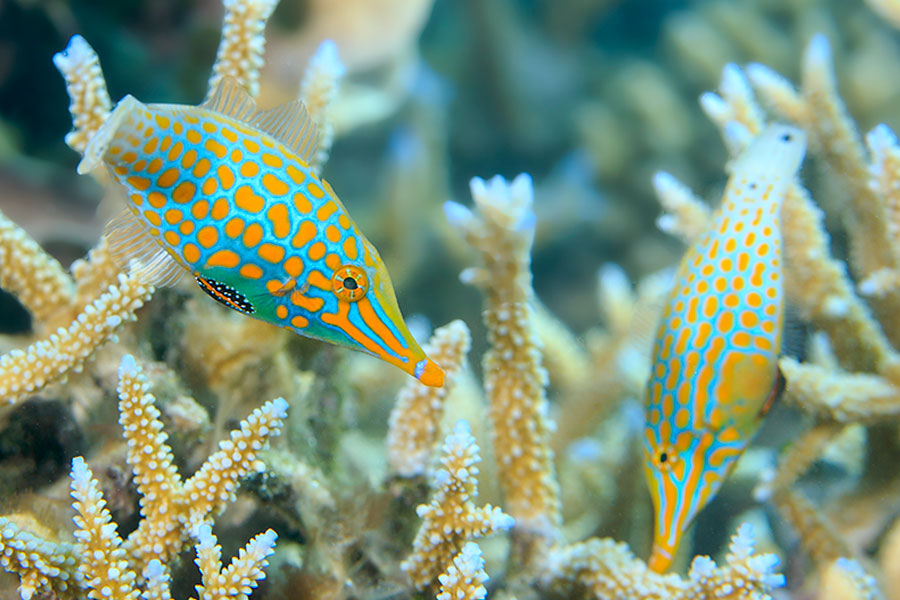This underwater image, likely taken in an ocean, sea, or possibly an aquarium, features two strikingly similar fish swimming amidst various aquatic organisms and coral-like structures. The fish, whose bodies are a vibrant turquoise blue, display distinct patterns of orange-yellow spots and stripes. Their long snouts and large eyes, with concentric circles of yellow and blue around a black center, add to their unique appearance. The fish on the left particularly stands out with its additional yellow markings and a notable black-and-white spotted fin. Surrounding the fish are brown, plant-like organisms with white spots, adding to the rich, albeit slightly blurry, backdrop of marine life.